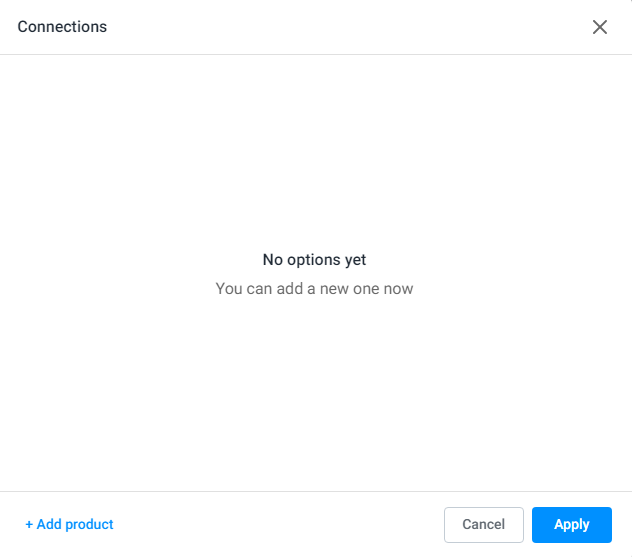A user interface screen displays an attempt to establish a connection, though the specific nature—whether to a person or a product—is unclear. The background is predominantly white, with the central message, "No options yet," emphasized in bold text. At the top left corner, the screen is labeled "Connections," with an 'X' button situated across from it, allowing users to exit. Below the main message, in the bottom left corner, a blue "+" symbol accompanied by the text "Add Product" is available, suggesting the option to add new items. Opposite, in the bottom right corner, there are two buttons: a white "Cancel" button and a blue "Apply" button with white lettering. The screen's layout is minimalistic and straightforward, though it lacks contextual information about the specific purpose of the connections, hinting at a possible functionality related to products or professional video conferencing.